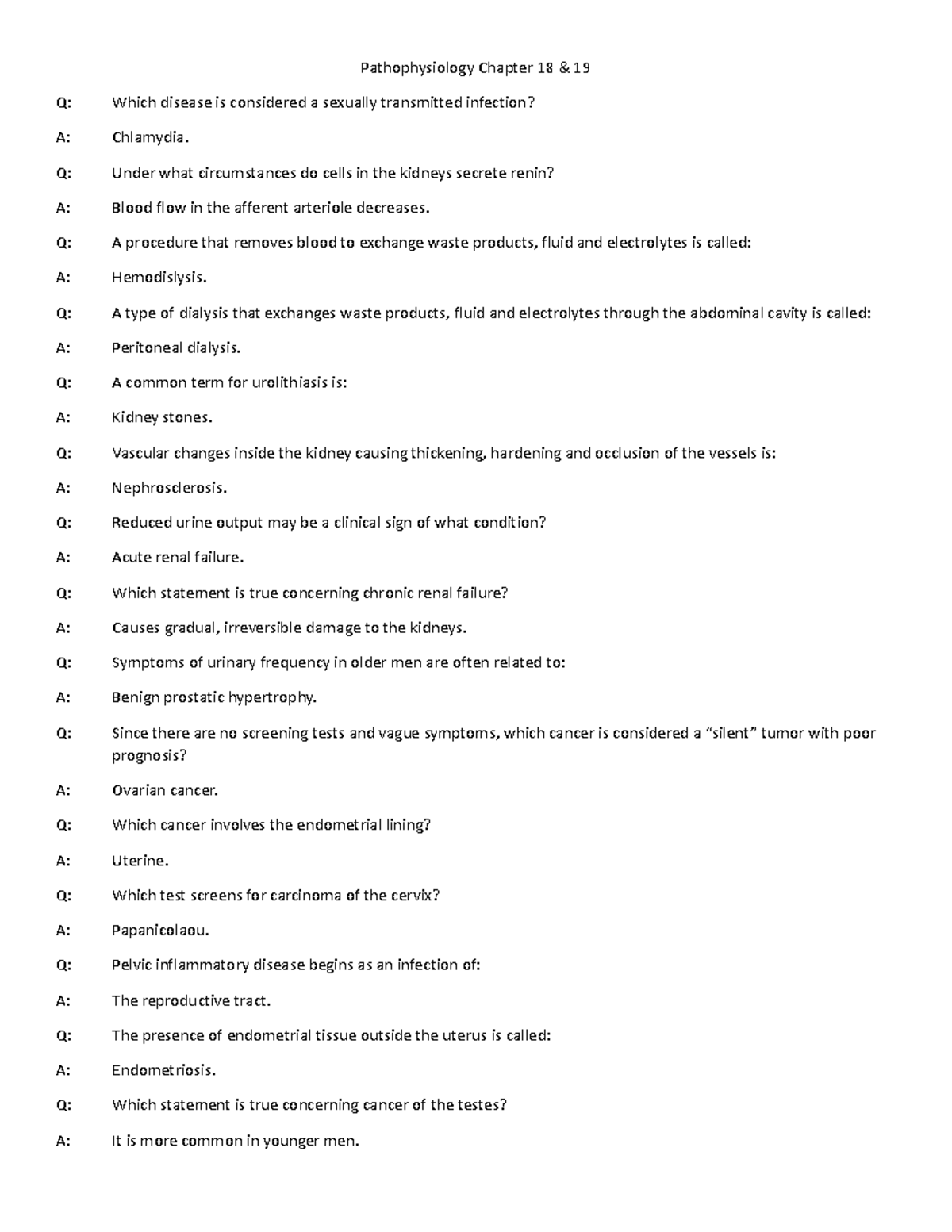This image depicts a page from a pathophysiology textbook, specifically from Chapters 18 and 19. The page is filled with a series of formatted questions and answers that cover various medical conditions and terminologies associated with pathophysiology. There are no graphics or photographs on this page; it solely consists of text. 

The content is structured with a "Q" preceding each question and an "A" preceding each answer. Some examples of the questions and answers on the page include:

- **Q:** Which disease is considered a sexually transmitted infection?
  **A:** Chlamydia.

- **Q:** A common term for urolithiasis is?
  **A:** Kidney stones.

- **Q:** Reduced urine output may be a clinical sign of what condition?
  **A:** Acute renal failure.

- **Q:** Symptoms of urinary frequency in older men are often related to?
  **A:** Benign prostatic hypertrophy.

- **Q:** Since there are no screening tests and vague symptoms, what cancer is considered a silent tumor with poor prognosis?
  **A:** Ovarian cancer.

- **Q:** Pelvic inflammatory disease begins as an infection of?
  **A:** The reproductive tract.

- **Q:** Which statement is true concerning cancer of the testes?
  **A:** It is more common in younger men.

The format and organization of the page suggest it is meant to test the reader's knowledge or provide a quick-reference review of important pathophysiological concepts.